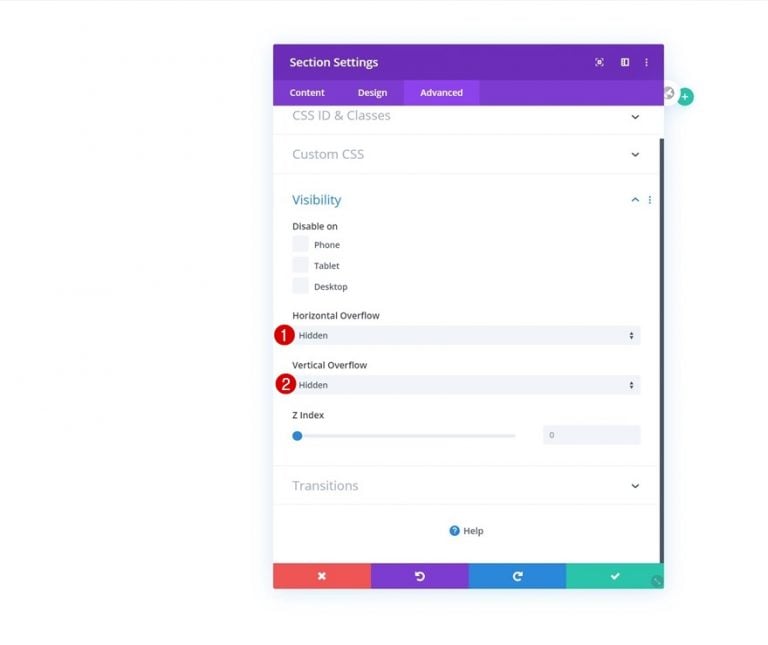The image displays a section settings screen on a device, set against a primarily white background with distinctive purple bands at the top and bottom. In the top purple band, "Section Settings" is prominently displayed in white text. To the right, there are three icons: a menu symbol represented by three vertical dots, what appears to be a QR code scanner, and another unclear icon.

The second purple section is divided into three categories: "Content," "Design," and "Advanced," with the "Advanced" category currently selected and displayed. Below this, several setting options are present. The "CSS ID & Classes" and "Custom CSS" subsections are both closed. The "Visibility" subsection is open and includes options to disable elements on phone, tablet, and desktop, though none of these are selected. This section also features "Horizontal Overflow" and "Vertical Overflow," marked by large red circles with the numbers 1 and 2, respectively.

Further down, the "Z Index" setting is visible and includes a scrollable bar set to the far left. The subsequent "Transitions" section is closed. Toward the bottom center of the screen, a help icon—a blue circle with a white question mark—offers assistance.

At the very bottom of the screen, there are four colored boxes with different icons: a red box with a white X, a purple box with a back symbol, a blue box with a forward symbol, and a green box with a check mark.